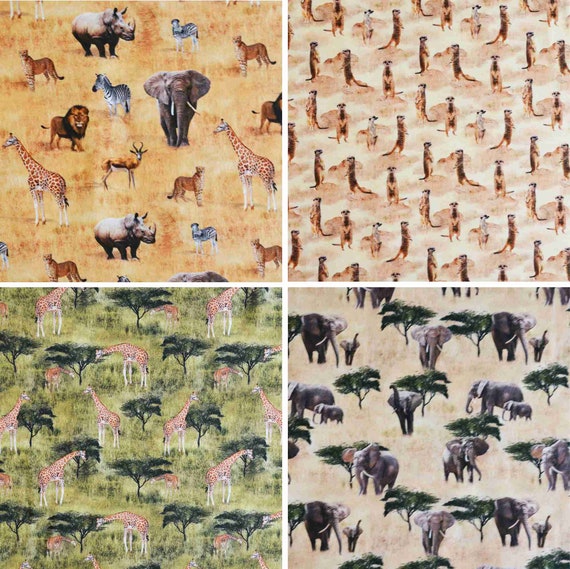This artwork is a hand-drawn or painted collage showcasing four detailed frames of African safari scenes, each teeming with a variety of animals. The top left frame features a diverse array of wildlife, including elephants, zebras, rhinos, cheetahs, lions, giraffes, hyenas, and antelopes, all standing on a backdrop of golden grass. The top right frame is dedicated to a group of about 20 meerkats, each facing different directions. In the bottom left frame, giraffes are depicted either standing in a field or eating from distinctive, bonsai-like trees, all set against a green backdrop. The bottom right frame highlights both adult and baby elephants navigating a landscape dotted with similar bonsai-like trees, with the animals rendered in color against a predominantly white background. This collage, evocative of vivid wallpaper or book illustrations, harmoniously blends these four scenes into one piece of art, celebrating the diverse wildlife and landscapes of Africa.